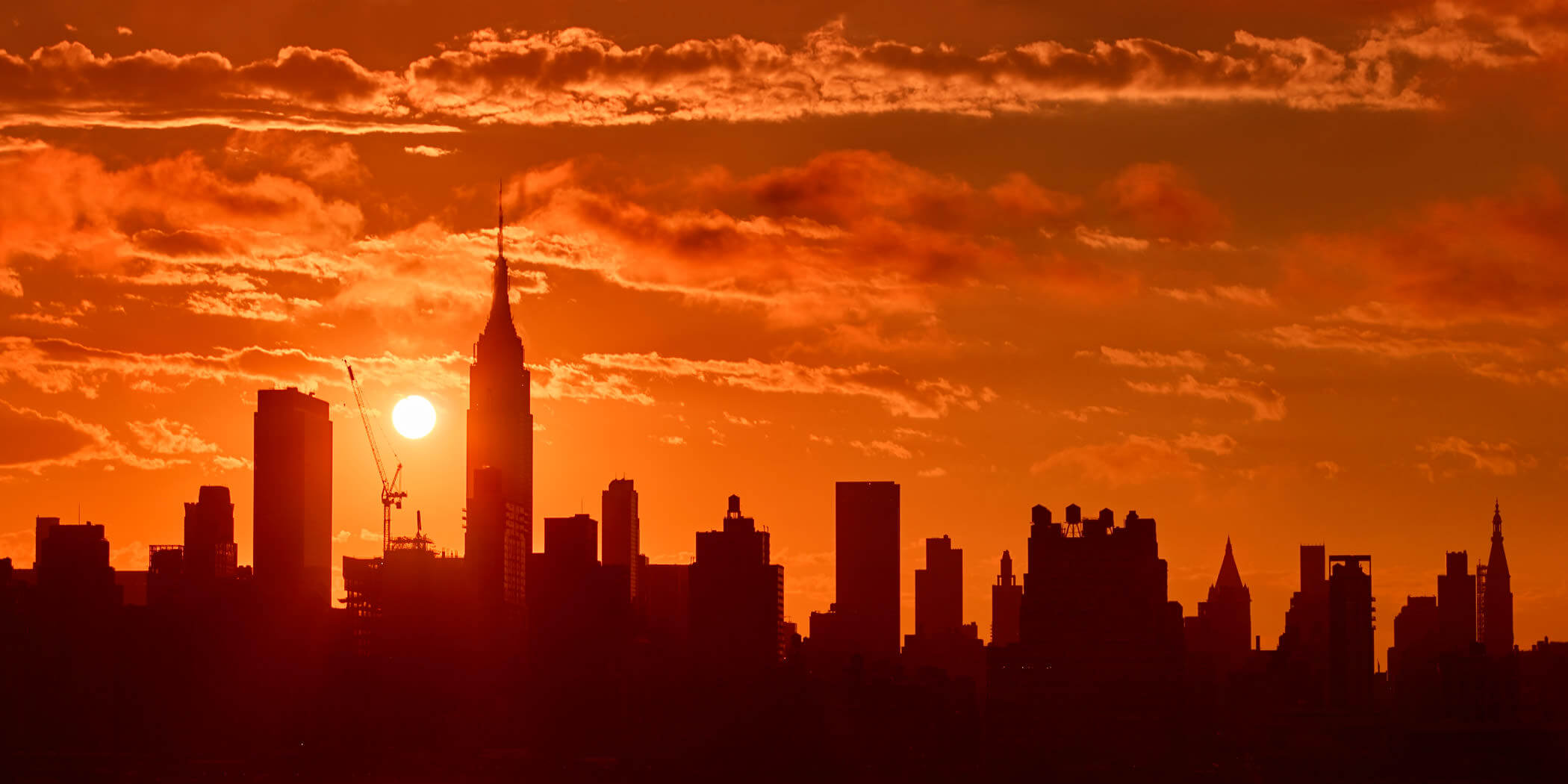A vibrant image captures a city skyline in silhouette during either sunset or sunrise. The high-rise buildings, painted in dark hues of brown and black, stretch across the horizon in a panoramic style. They begin small on the edges and rise to a peak around a quarter of the way into the frame, where a prominent crane is also visible standing next to the tallest skyscraper. The sun, a blazing and blinding sphere of bright yellow, sits just above the crane, casting a dramatic backlight on the scene. The sky is a striking tapestry of multi-shaded orange and brown, with touches of tan and yellow. Puffy clouds streak across from left to right, varying from dark gray at the top to bright orange at their bases, reflecting the sun's intense glow. The entire composition creates a mesmerizing contrast between the darkened cityscape and the bright, dynamic sky, encapsulating the beauty of a bustling metropolis at the day's edge.